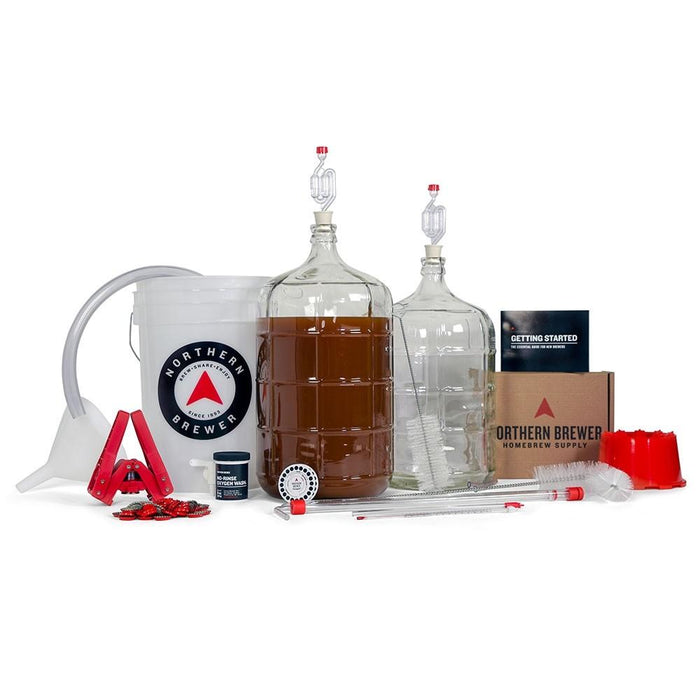This photograph displays a detailed beer brewing starter kit branded Northern Brewer. At the center, two large bottles are prominently featured: one clear with a bottle brush inside it, and the other filled with an amber-colored liquid. To the left, a white bucket with a blue and red emblem and the Northern Brewer logo stands equipped with a funnel and various pieces of equipment including a bristle brush and a long tube. Additional red clamps, tubes, and a metallic bristle brush are scattered across the front. On the right, a brown cardboard box and a black booklet labeled “Getting Started” are visible, alongside the Northern Brewer Home Brew Supply branding. Other brewing apparatus such as airlocks, a bottle cap machine, and siphons complete the setup, indicating this comprehensive collection is intended for crafting homemade alcoholic beverages.